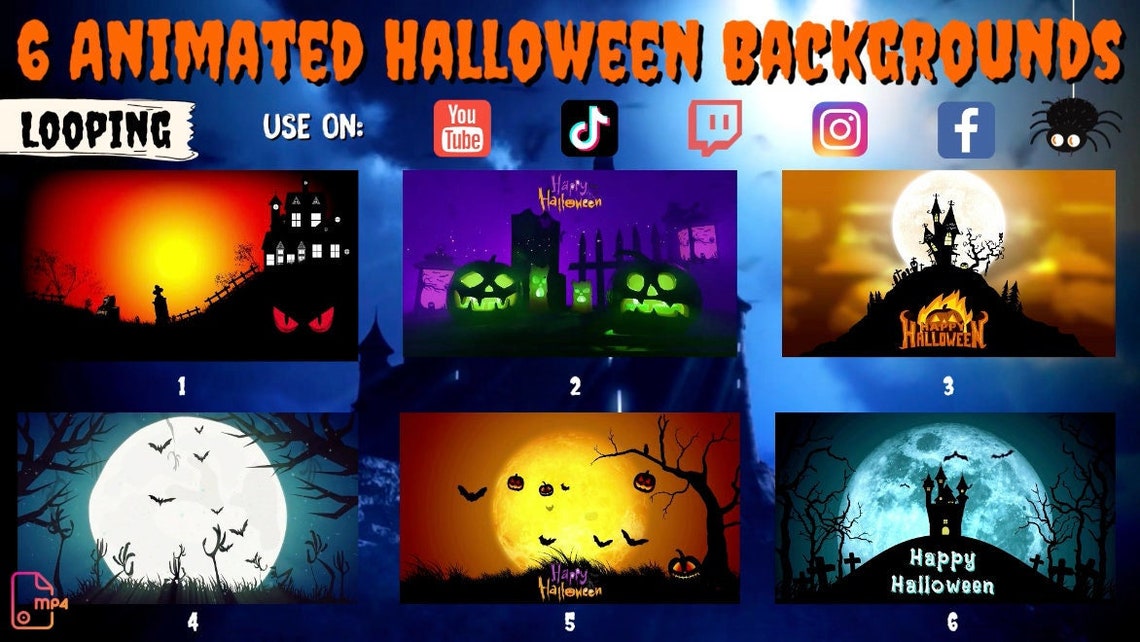This screenshot captures a website featuring a selection of automated Halloween-themed backgrounds designed for social media profiles. The background of the website is a captivating night scene in shades of blue, lending a spooky atmosphere. At the top, vibrant orange text prominently displays "Automated Halloween Backgrounds," with a subtitle below that reads "Use on" followed by icons for YouTube, TikTok, Twitch, Instagram, and Facebook, indicating compatibility with these platforms.

Six rectangular backgrounds are showcased on the page, each aligning with the Halloween theme in distinct yet eerie ways. The top left background portrays a night scene drenched in hues of orange and red, fading into a sinister black in the lower right corner, where eerie red eyes lurk in the darkness. The center image on the top row contains jack-o'-lanterns, uniquely green instead of the traditional orange, adding an unusual twist to the familiar visage. The top right background features an ominous haunted house perched atop a hill, backlit by the glow of a full moon.

The three backgrounds on the bottom row are unified by the presence of a large, bright full moon. The bottom left includes traditional Halloween elements, while the bottom center combines various spooky visuals. The bottom right background prominently displays the message "Happy Halloween," enhanced by the haunting luminescence of the full moon.